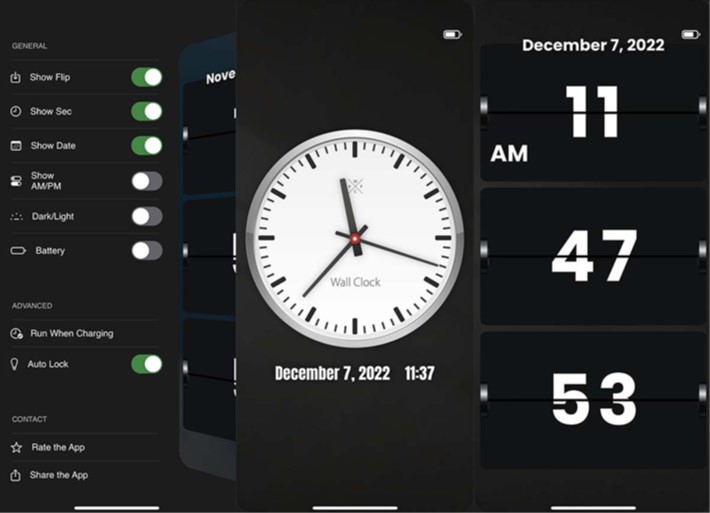The image comprises a series of three distinct, portrait-oriented screens arranged against a black backdrop, providing an intricate and somewhat confusing visual experience. The overall image is slightly taller than it is wide.

1. **Leftmost Image:** This screen showcases a settings menu with a black background and a white header labeled "General." The menu lists six options with toggle switches: "Show Flip," "Show Sec," "Show Date," "Show AM/PM," "Dark Light," and "Battery." The first three toggles are switched on, indicated by their green colors. Below these options, the "Advanced" section includes settings like "Run when Charging" and "Autolock," with "Autolock" switched on. Further down, options for "Contact," "Rate app," and "Share this app" are displayed.

2. **Middle Image:** This screen displays an analog wall clock with a simple and clean design. The clock has a white background and a gray frame, showing a time that is approximately 11:37. The ceiling and floor of the clock face are both white, contrasting with the black background.

3. **Rightmost Image:** This screen shows a digital clock app with a flip-style display. The app indicates a time of 11:47 and 53 seconds, which is different from the time displayed on the analog clock. This flip clock display also features a battery icon positioned on a different part of the screen compared to the settings and the analog clock images, suggesting these are separate screens consolidated into one image.

Overall, the composite image, though appearing as a single unit, is a collection of three separately detailed visuals highlighting different time-related displays and settings on digital devices.